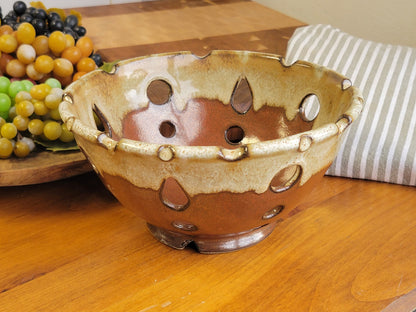The image depicts a meticulously decorated scene centered around a handmade stoneware bowl on a warm yellowish wooden table. The bowl, positioned prominently in the center, features a rich red-brown base with a creamy beige glaze that drips down from the top, adding depth to its textured appearance. The bowl has numerous teardrop-shaped cutouts that suggest it is more decorative than functional. To its left, a wooden dish holds an assortment of vibrant plastic grapes in shades of black, brown, green, and yellow, adding a touch of color to the scene. Meanwhile, to the right of the bowl, a folded striped napkin in alternating white and grayish-tan hues lies neatly on the table. The background is set against a cream-colored wall and includes a cutting board with varied wooden hues, contributing to the warm and inviting atmosphere of what appears to be a dining room area. A gray and white pillow or cushion can be glimpsed in the back right, enhancing the cozy, homey vibe of the setting.